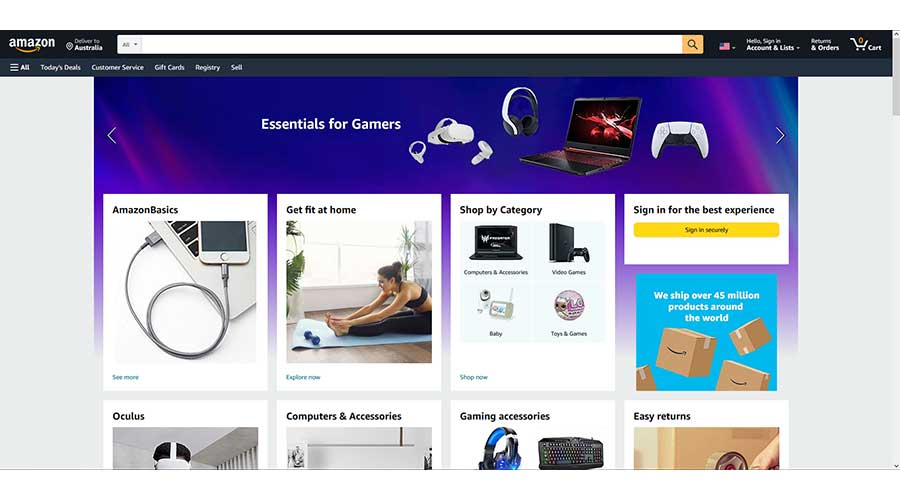This image is a screenshot of an Amazon webpage, captured on a user account with delivery set to Australia. The top of the screen features a thin black navigation bar with the Amazon logo on the left, displaying the iconic white text and the arrow that resembles a smile. Just to the right of the logo, it reads 'Deliver to Australia.'

Prominently centered below the navigation bar is a large, white search box that allows users to enter search queries. The search box includes a search icon on one side and a dropdown menu for selecting specific categories on the other. Adjacent to the search box, there is a small flag, possibly representing the United States, displaying red, black, and white colors, although its exact identification is unclear.

Further up on the navigation bar, users can find additional links for returns and account information.

The webpage itself is currently displaying a feature section titled "Essential for Gamers," highlighting various gaming-related products. This section includes images of a laptop, what appears to be a VR device, headphones, and other gaming accessories.

Below this are distinct sections for different categories such as 'Amazon Basics,' 'Get Fit at Home,' and 'Shop by Category,' each accompanied by relevant images to help guide users. The website's primary color theme transitions from purple at the top to white, with text and images neatly organized in individual boxes underneath.